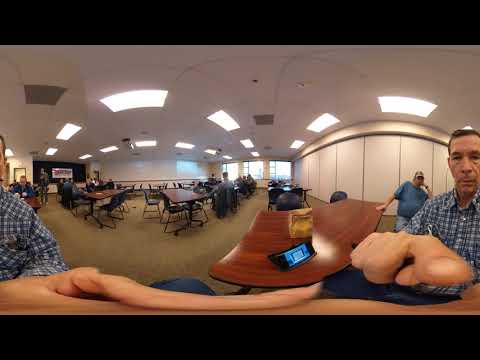This panoramic image captures a bustling indoor conference room, possibly a convention or large meeting space, characterized by its tan-colored floor, paneled white walls, and trio of distant windows. The ceiling features bright, rectangular fluorescent lights, which appear rounded due to the panoramic effect. The room is furnished with several long tables and benches, mostly unoccupied, but a few with attendees. 

In the foreground, a middle-aged Caucasian man with thinning hair and a gaunt build is activating the camera with his hand visible due to the panoramic view. He is dressed in a blue and white plaid button-up shirt. Next to him, a heavyset man in a baseball cap and blue t-shirt, paired with jeans, is seated. They appear to be sitting at a wooden desk that has a tablet or phone and a paper sack lunch on it. 

The background of the room features a black wall adorned with a banner, though the text is unreadable due to the image's low resolution. Near this wall, a figure appears to be speaking into a microphone, reinforcing the notion that the setting is a formal gathering space, likely within a hotel or visitor's center.